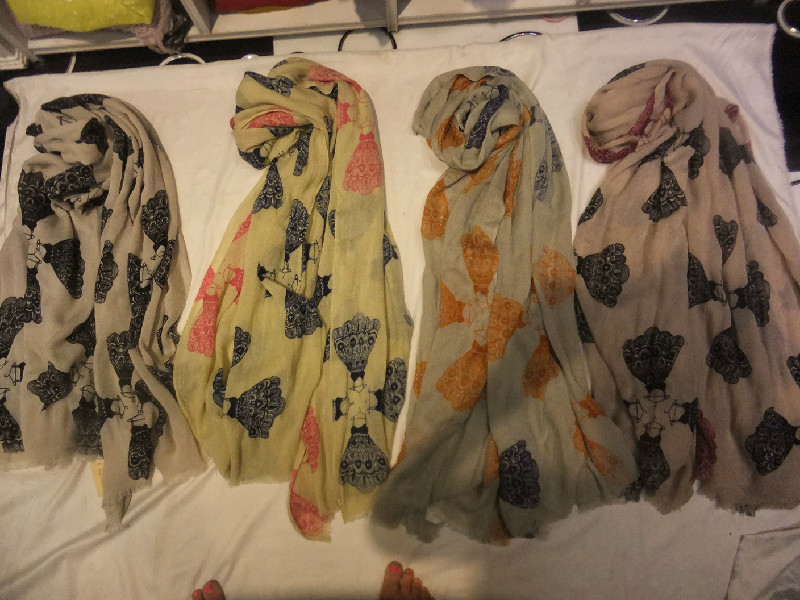The photograph captures an indoor scene with four distinct shawls or scarves, artfully arranged on a white fabric background. From left to right, the first shawl features a white background adorned with black symbols. Next is a vibrant yellow shawl embellished with red and black symbols. The third shawl showcases a light greenish-gray hue with yellow and black designs. Finally, the fourth shawl is a very light pink adorned with black and subtle red details. The setting appears to be a small cubby or bay, separated by thin white shelves. Additionally, at the bottom of the image, the feet of a woman with red or orange nail polish on her toes are visible, indicating her presence as the likely photographer.